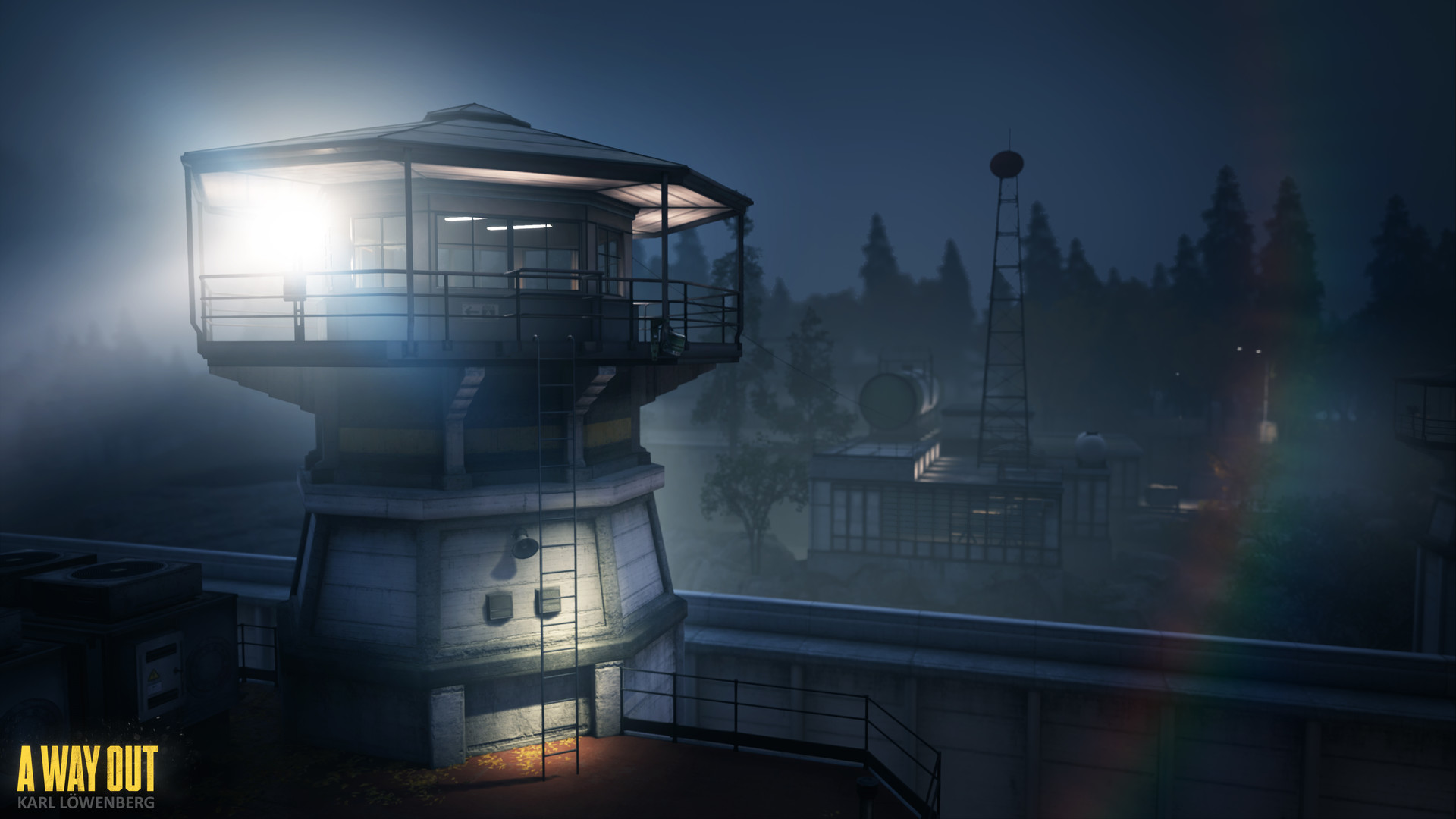The image depicts a dark, nighttime scene featuring a brightly lit watchtower or security tower with a metal ladder running up its side. At the top of the tower, there's a railing surrounding the exterior, and windows offer a glimpse into the illuminated interior. The sky is dark with hints of light possibly originating from the tower itself. A building with a large satellite dish is visible in the background, and additional structures, including what appears to be a water tower, can be seen to the right of the main tower. Trees, likely evergreens, populate the distant background. In the lower left corner, the image is captioned with "A Way Out" in bright yellow capital letters, followed by the name "Karl Lowenberg." The overall composition suggests a scene from a book cover, movie, or video game, presenting an atmospheric and somewhat mysterious outdoor setting.